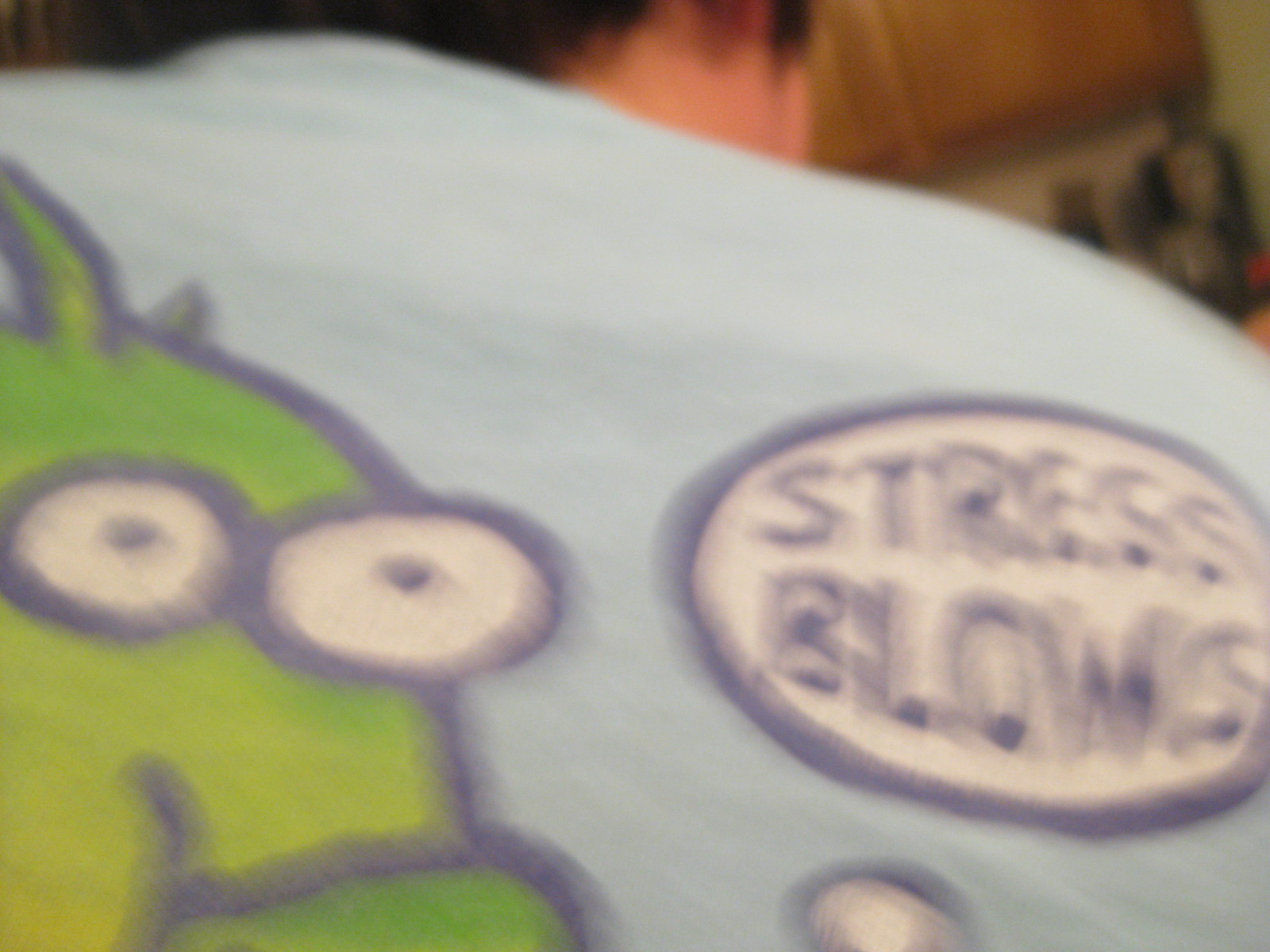An action shot features the back of a man in motion, resulting in a blurry image. The man is wearing a light blue shirt adorned with a whimsical, green monster-like creature on the left side, characterized by its large round eyes and neutral expression, accented by yellow highlights. On the right side of the shirt, there's a speech bubble with the words "STRESS BLOWS" in all caps, though the text is difficult to read due to the blurriness. The man, who has close-cropped dark brown hair and pale skin, is seen slightly from behind, looking away from the camera. The background reveals light brown cupboards, several bottles, and a counter surface, all set against an off-white wall.